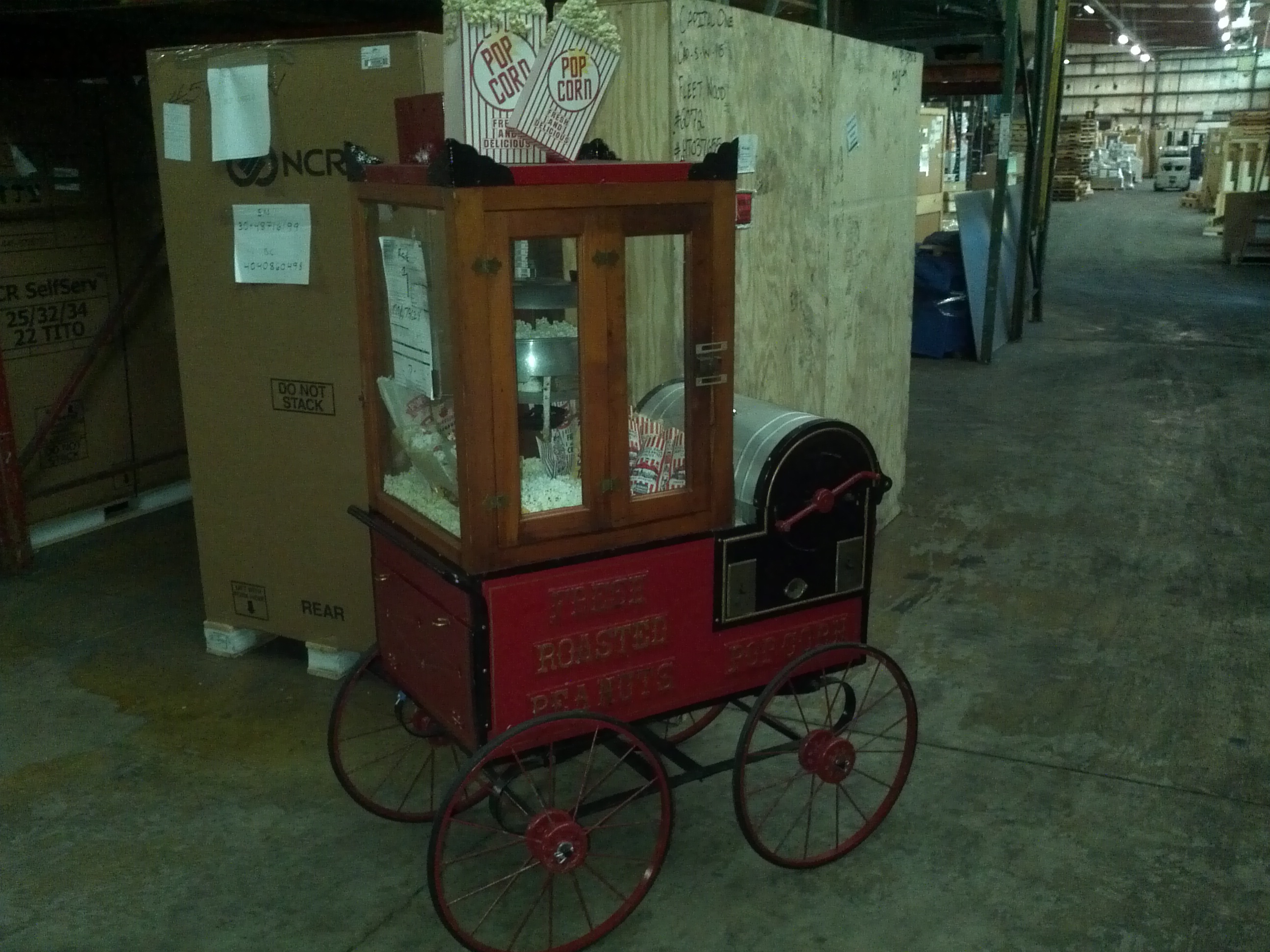In a large, somewhat cluttered warehouse, a small, charming popcorn cart stands prominently. The cart, painted in bright red, features large, dark brown wheels reminiscent of wagon wheels, complete with visible spokes. Despite prominently displaying "Roasted Peanuts," the cart is adorned with red and white striped containers filled with yellow corn kernels, indicating its primary use for popcorn. At the top, a wooden cabinet houses a traditional metal popcorn popper. Around the cart, various packages and a large brown cardboard box suggest a recently abandoned setup. The background shows an array of other vendor setups, hinting at a bustling, albeit currently quiet, vendor area.